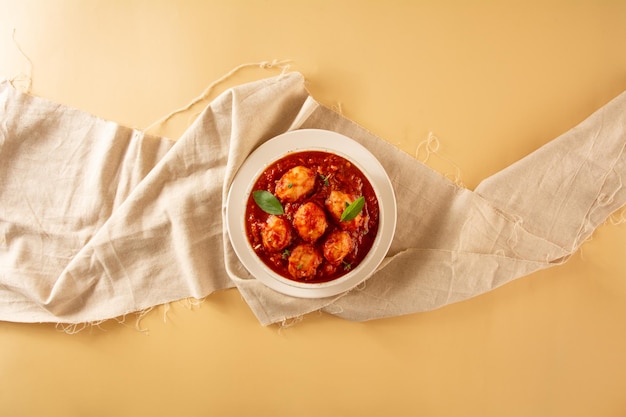This photograph captures a meticulously arranged meal from an aerial perspective. The background features a slightly illuminated, gradient mustard yellow surface with a large, thick strip of undyed linen or muslin fabric horizontally spread across. The fabric, appearing somewhat crumpled, is thicker on the left and thinner on the right, folding up and back down around the center. Resting atop this linen is a plain white ceramic or earthenware dish holding a bowl of food. 

Inside the white bowl lies a rich, bright red tomato-based sauce, accentuated with six evenly spaced meatballs or similar spherical items, positioned with two at the bottom, two on the sides, one in the center, and one on top. Garnishing this dish are two green leaves, possibly mint or basil—one placed between two meatballs in the top left and the other topping the right-hand meatball. Additional finely chopped herbs sprinkle the dish, adding a touch of freshness and contrast to the deep red sauce. The setting and simple, yet elegant presentation suggest that this is a home-cooked meal ready to be shared.